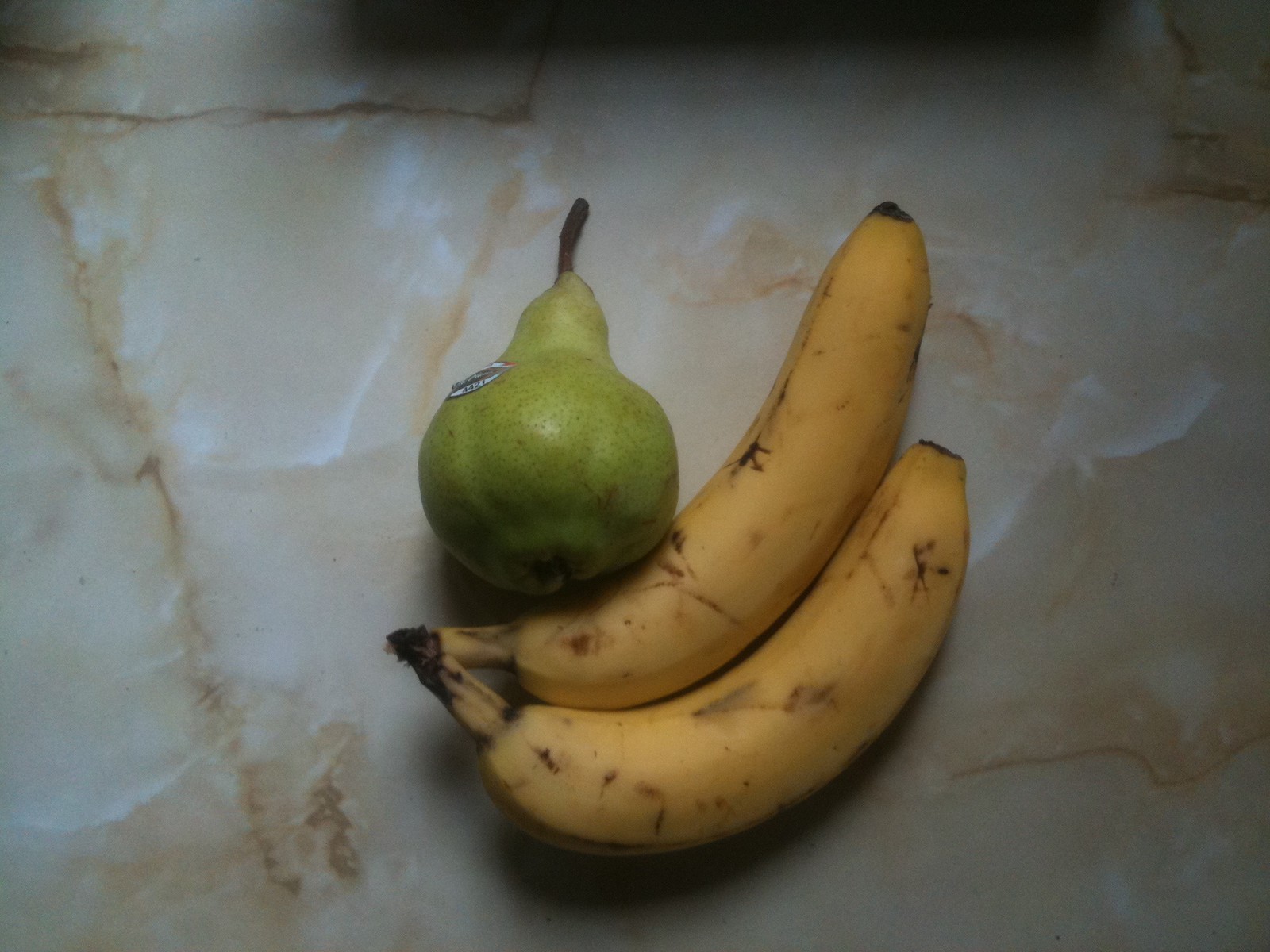This color photograph showcases a still life composition of two bananas and a pear artfully arranged on a pristine white marbled surface. The pear, positioned at the top of the frame, exhibits a gradient of green hues, transitioning from a light green at its upper portion to a darker shade towards its base. Its woody stem protrudes from the top, adding to its natural charm. A produce label is affixed to the pear's left side, though it remains illegible. Subtle browning at the bottom of the pear hints at natural ripening. The pear is slightly tilted, resting against one of the bananas.

Below the pear, two bananas are still attached at their stems, forming a graceful upward curve towards the right. The intersection where the stems meet is distinctly brown, indicative of their harvest. The bananas' skins are predominantly yellow, speckled with numerous brown spots, showcasing their ripeness.

The photograph is landscape-oriented, wider than it is tall, ensuring the focal subjects are comfortably spread across the frame. There are no people, animals, plants, flowers, trees, buildings, billboards, signs, or motorized vehicles present in this serene and minimalist composition.